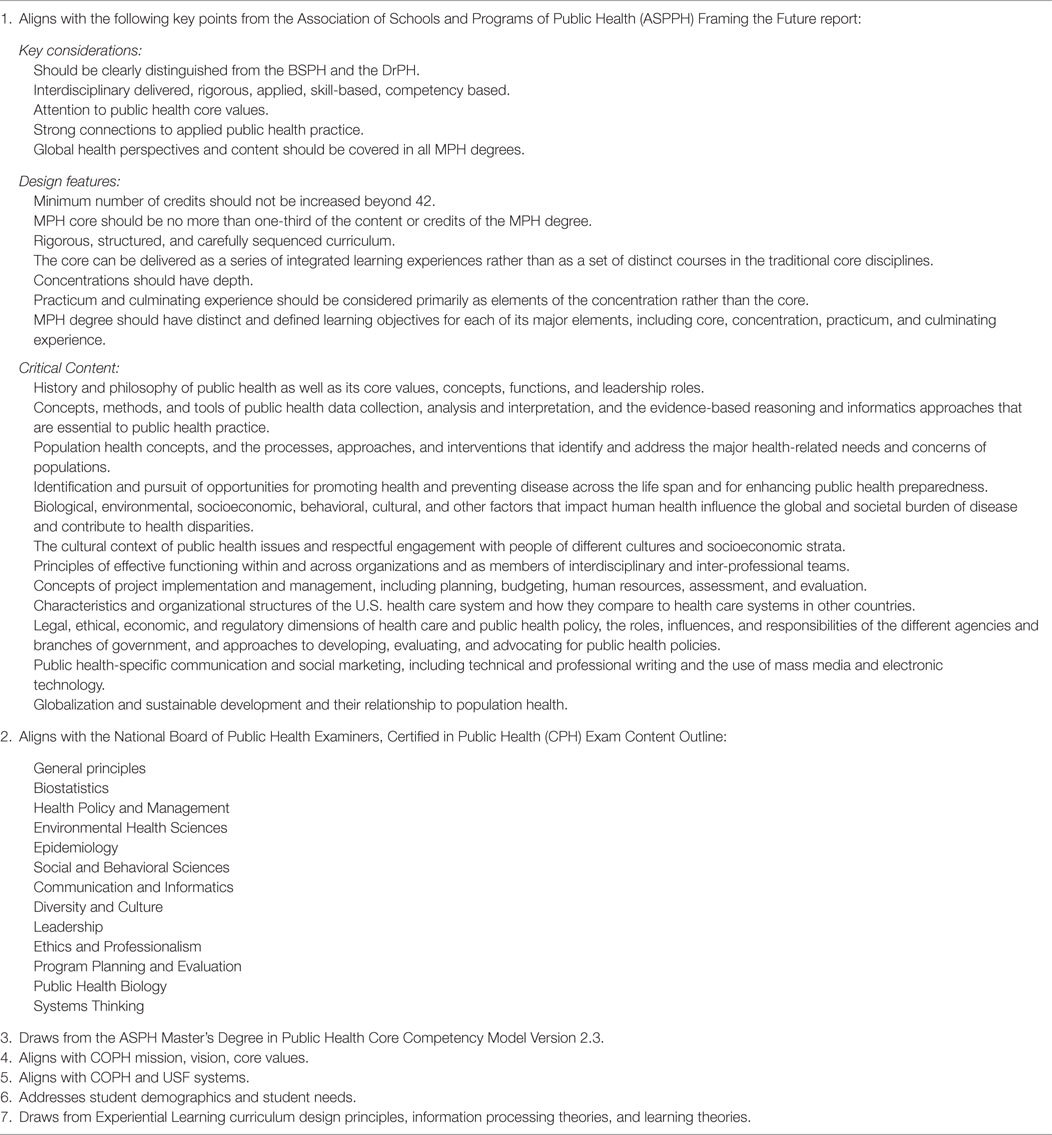**Detailed Caption:**

The image features a white background with small black text. At the top, a title reads, "Number One: Aligns with the Following Key Points from the Association of Schools and Programs of Public Health (ASPPH) Framing the Future Report." Below the title, several sections detail key considerations, design features, critical content, and alignments with standards relevant to public health education.

**Key Considerations:**

- Distinguishing characteristics between the BSPH (Bachelor of Science in Public Health) and DrPH (Doctor of Public Health) programs.
- Emphasis on an interdisciplinary, delivered, rigorous, applied, skill-based, and competency-based curriculum.
- Focus on public health core values and strong connections to applied public health practice.
- Inclusion of global health perspectives and content in all MPH (Master of Public Health) degrees.

**Design Features:**

1. The minimum number of credits should not exceed 42.
2. The MPH core should comprise no more than one-third of the total content or credits.
3. A rigorous, structured, and carefully sequenced curriculum should be in place.
4. The core can be delivered via integrated learning experiences instead of distinct courses.
5. Concentrations should have depth.
6. Practicum and culminating experiences should primarily be elements of the concentration rather than the core.
7. The MPH degree should have clearly defined learning objectives for the core, concentration, practicum, and culminating experiences.

**Critical Content:**

1. General Principles
2. Biostatistics
3. Health Policy and Management
4. Environmental Health Sciences
5. Epidemiology
6. Social and Behavioral Sciences
7. Communication and Informatics
8. Diversity and Culture
9. Leadership
10. Ethics and Professionalism
11. Program Planning and Evaluation
12. Public Health Biology
13. Systems Thinking

**Additional Alignments:**

- Number Two: Aligns with the National Board of Public Health Examiners (NBPHE) Certified in Public Health (CPH) exam content outline.
- Lists the same critical content with emphasis on competencies required in public health certification exams.
- Number Three through Seven outline further alignments:
  - Number Three: Draws from the ASPH Master's Degree in Public Health Core Competency Model Version 2.3.
  - Number Four: Aligns with the COPH (College of Public Health) mission, vision, and core values.
  - Number Five: Aligns with COPH and USF (University of South Florida) systems.
  - Number Six: Addresses student demographics and student needs.
  - Number Seven: Draws from experiential learning curriculum design principles, information processing theories, and learning theories.

A fine grey line runs horizontally across the bottom of the text, separating these detailed points from any subsequent content.